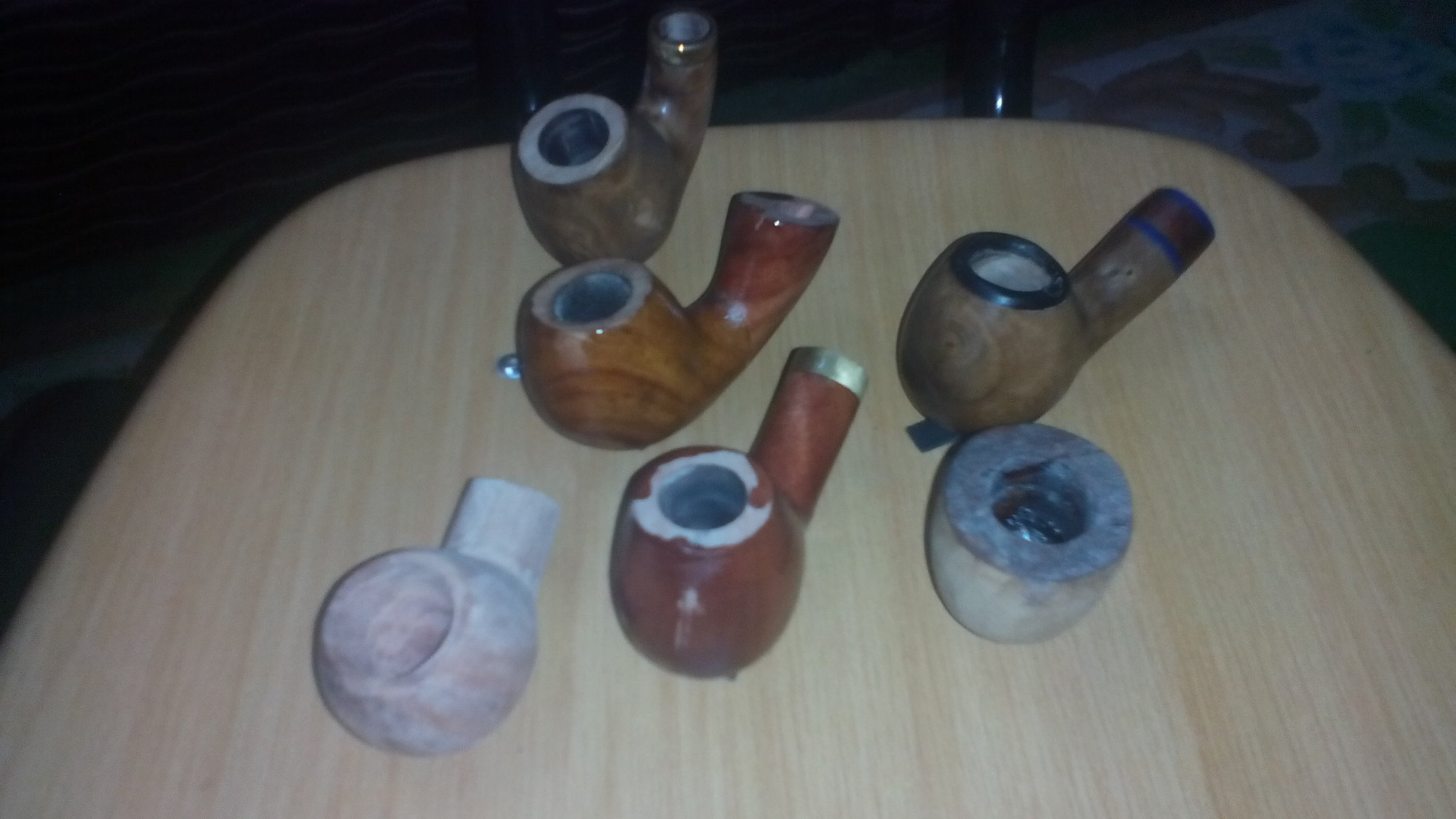This is a color photograph, albeit not very well-lit, showcasing six short-stemmed pipes seated on a pale woodgrain chair with a curved edge towards the back. The front edge of the chair is not visible. The pipes, arranged in a variety of materials and colors, rest face-up with their bowls prominent. 

Distinctive features about the pipes include their varying compositions: some appear to be intricately carved out of different wood grains, like one with a light-medium brown color, while another has a metal tip for inhaling smoke. There's also a smaller pipe, seemingly made of stone and a larger, mossy green one that also appears to be stone-carved. Additionally, a grayish-white ceramic pipe, a maroon-colored set, and a blue-rimmed gray bowl pipe are part of the collection.

The flash reflection highlights parts of the scene, and beyond the chair, in the dark shadows, lies a patterned carpet that subtly adds depth to the photograph.